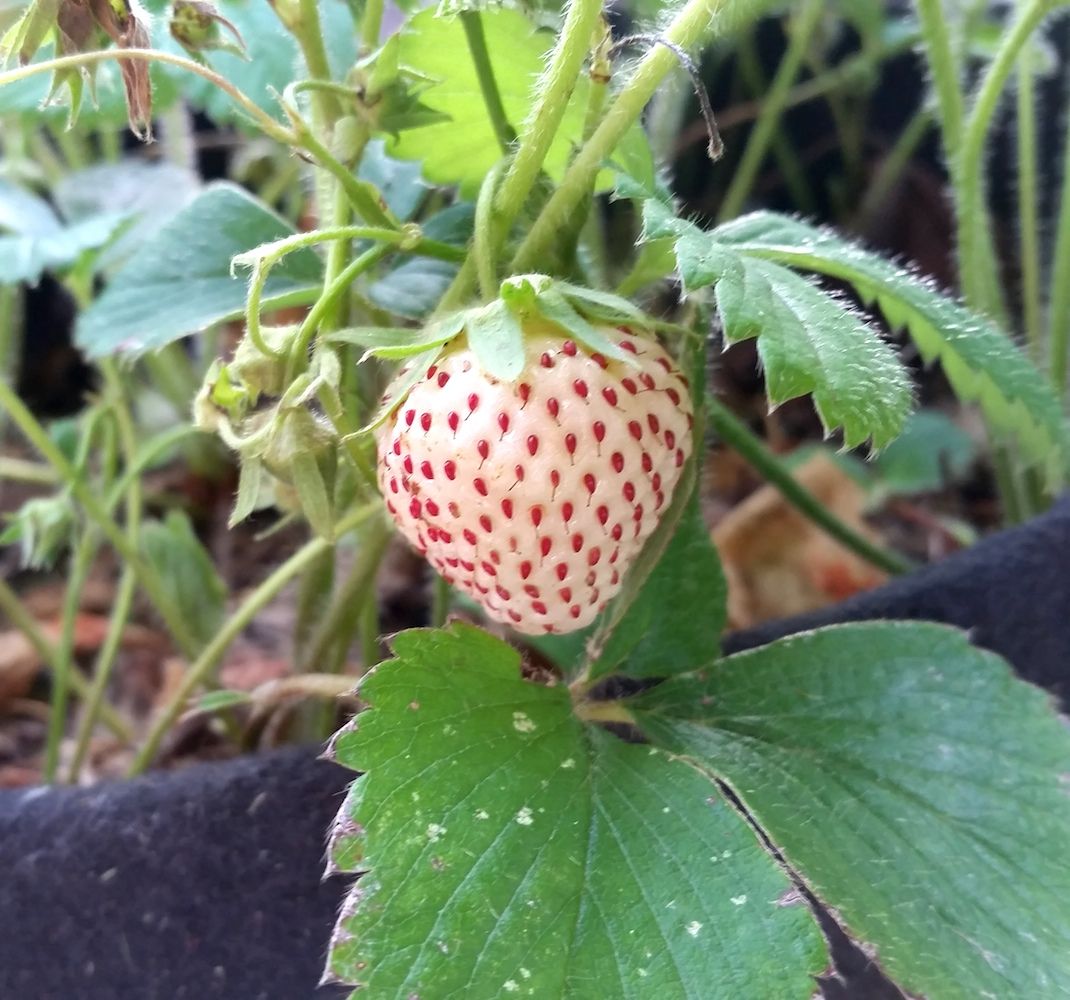This is a very close-up and professionally taken photograph of a single, unripe strawberry centered on a strawberry plant. The strawberry itself is fairly large but predominantly white with numerous red spots indicating its immature stage, possibly a week or two from ripeness. The seeds, noticeable for their red color, appear to have tiny black micro hairs attached. The plant's large green leaves, some speckled with white spots, frame the strawberry below, while smaller leaves and fuzzy, green stems extend above it. Encircling the bottom of the image is a black burlap sack, suggesting the plant is either growing in a pot or within a bordered garden bed. The background subtly showcases the natural garden environment with hints of other plants and colors like green, black, pink, red, and a touch of brown.